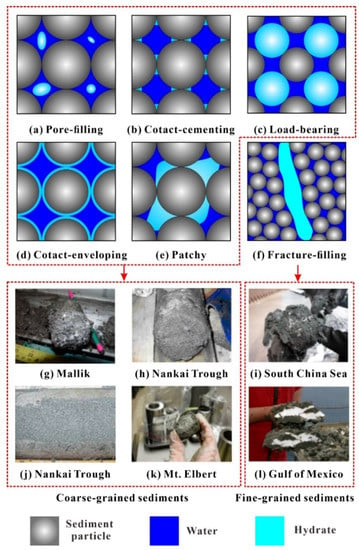The image is a highly detailed flowchart-style collage consisting of 12 squares, each displaying different diagrams illustrating molecular structures and sediment packing. At the top of the image, starting from the top right, are three boxes labeled as "pore-filling," "contact cementing," and "load-bearing," showing circular, sphere-like molecules in gray, blue, and light blue colors. The second row displays further variations labeled "contact enveloping," "patchy," and "fracture-filling."

The bottom section showcases six additional pictures representing different sediment descriptions. The first three are "Malik," "Nankai Trough," and "South China Sea," followed by another entry of "Nankai Trough," and finally "Mount Albert" and "Gulf of Mexico." This section is divided into coarse-grained sediments on the left and fine-grained sediments on the right. 

A color-coded legend at the bottom of the image provides clarity: "sediment particle" in gray, "water" in dark blue, and "hydrate" in light blue. This comprehensive set of diagrams effectively categorizes different types of sediments and their molecular interactions, providing a clear visual guide to their structural formations in various global locations.